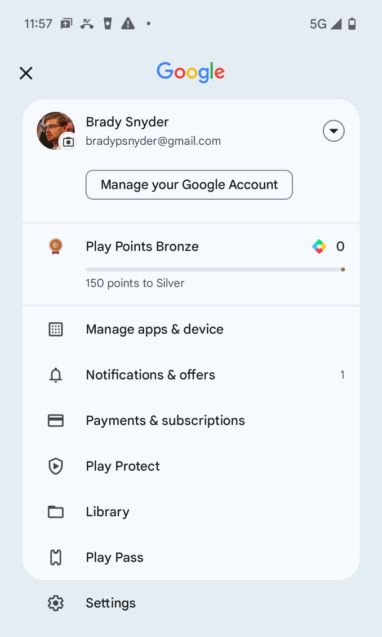The image displays a cell phone screen with the time "11:57" in the top-left corner. In the top-right corner, there are icons indicating a 5G connection, cellular reception, and battery status. Below this, the Google logo is visible with a small circular photo of a man to its left. Next to the photo, it reads "Brady P. Snyder at gmail.com."

Directly below this, a rectangular section contains the text "Manage your Google account." Further down, there's an icon resembling a prize ribbon, accompanied by the text "Play Points Bronze, 150 points to Silver." Following this is a square icon with dots inside it, labeled "Manage apps and device."

Further down, there's an image of a bell with the text "Notifications and offers." To its right, a "1" indicates there is one new notification. Below this, there's an icon resembling a payment card with the text "Payments and subscriptions" next to it. Underneath this is an icon of a badge with a play button, labeled "Play Protect."

Further down the screen, an icon of a folder appears next to the text "Library." This is followed by an icon resembling a movie ticket with the text "Play Pass" beside it. Finally, at the bottom, there's an icon of a gear with the label "Settings."

There are no additional images or text beneath the "Settings" section, marking the end of the content displayed on the page.